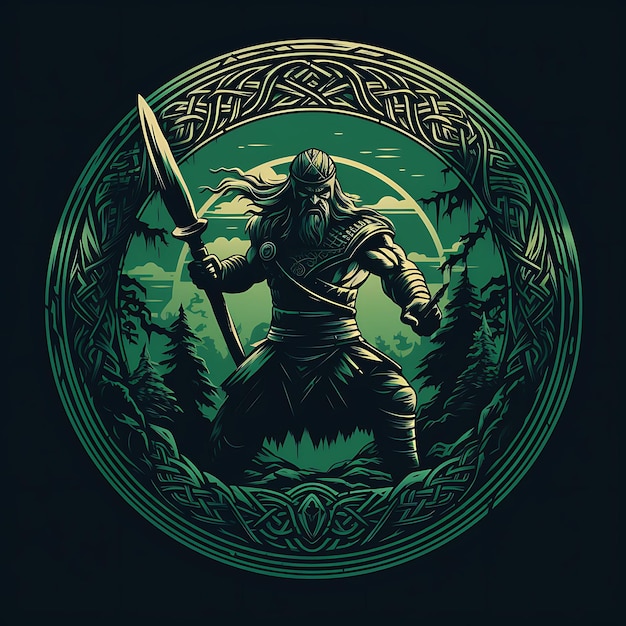In the image, set against a stark black background, a formidable warrior takes center stage. Dominating the scene is a large, round combat shield, meticulously adorned with intricate silver braids along its edges. The warrior, exuding an aura of intimidation, sports long, wind-swept hair that adds to his fierce demeanor. A headband secures his hair, drawing attention to his angrily intense eyes. His face is further accentuated by a thick beard and mustache that amplify his rugged appearance. The warrior's muscular frame is clad in imposing armor, emphasizing the broad expanse of his chest and powerful arms. A sturdy belt cinches his waist, complementing his overall rugged outfit. Clutched in his hand is not a sword, but a formidable spear, showcasing his readiness for battle. Enveloping him are shadowy trees, creating a dramatic backdrop that emphasizes his heavy, robust legs, completing the image of an indomitable warrior poised amidst the wilderness.